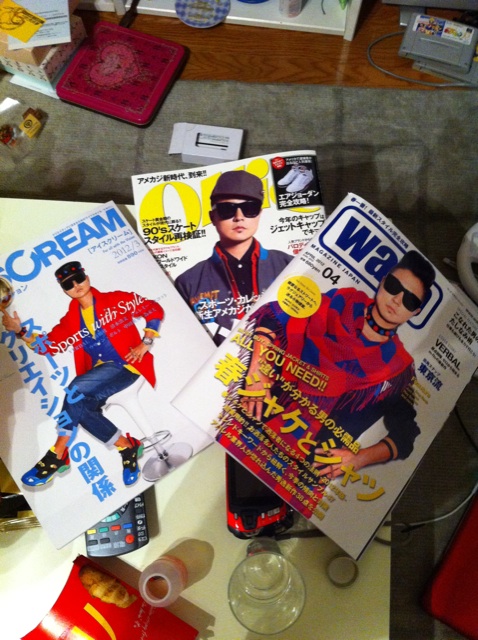In a cluttered room that resembles either a kid's or a college student's space, sits a yellow table laden with various items. The floor, possibly gray carpet, is strewn with a white cardboard box featuring a heart, some games, and other trash. On the yellow table, three different fashion or style magazines prominently display Asian men on their covers, all sporting sunglasses and wearing vibrant clothing like red and royal blue. One magazine is clearly titled "Cream," while the other two have partially legible titles starting with "O" and "W-A." These magazines are haphazardly arranged, with one partially covering a remote control. Scattered alongside them are a phone, a transparent glass, and an empty red McDonald's fries container. Japanese writing is visible on the magazines, contributing to the room's eclectic atmosphere.